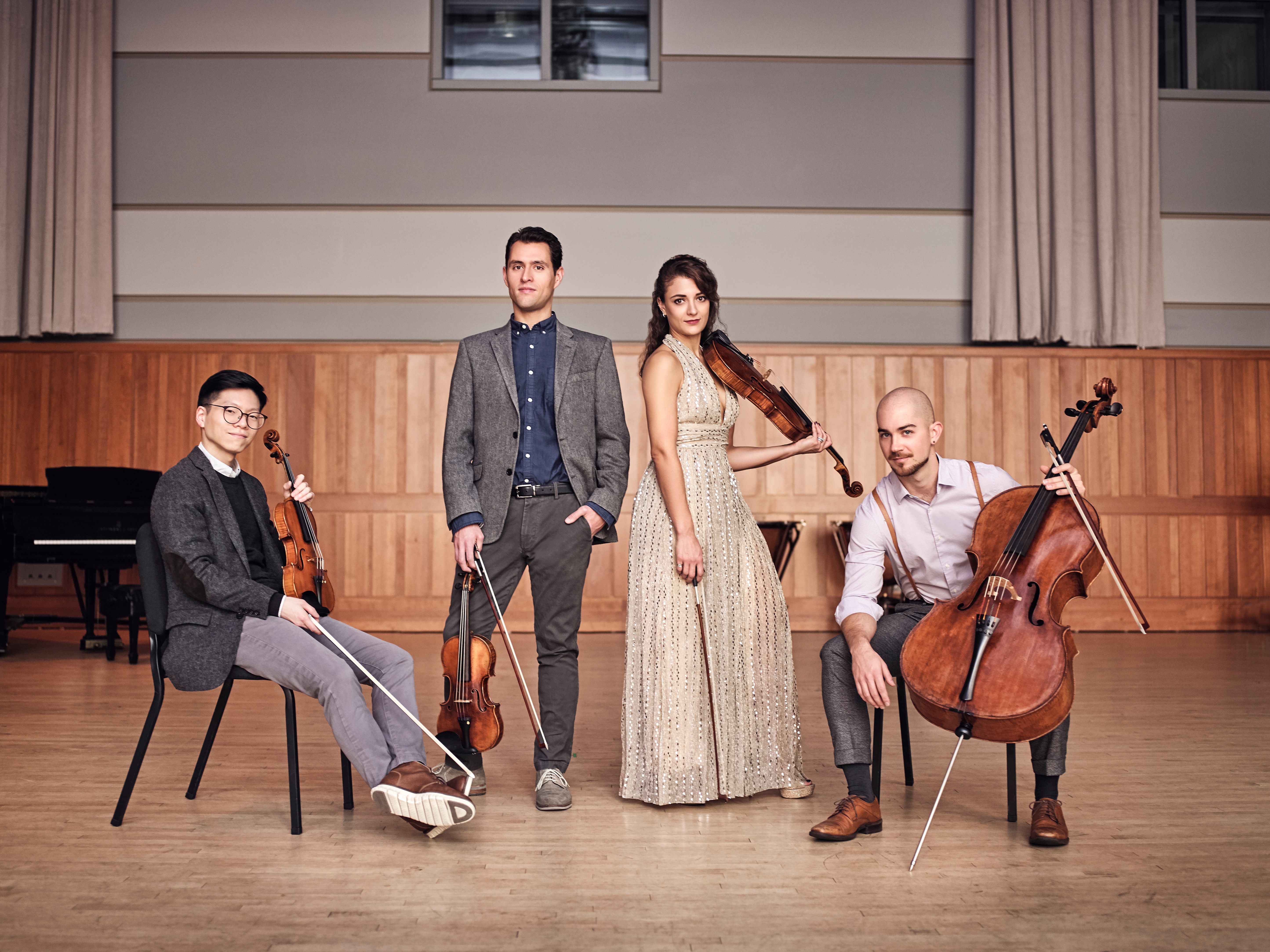This photograph captures a string quartet performing in a large indoor auditorium with distinctive, wood-paneled flooring and high ceilings. Seated on the far left is an Asian man wearing glasses, dressed in a jacket and pants, holding his violin and bow and resting his fingers on the fretboard. To his right stands another gentleman in a gray suit jacket with a blue shirt, casually holding his violin and bow in his right hand while his left hand rests in his pocket, suggesting a relaxed demeanor. Next to him, a striking woman in a stunning, gold, low-cut, sleeveless gown elegantly rests what appears to be a viola on her shoulder, with the bow poised in her right hand. Lastly, on the far right, a young, bald man with a beard, dressed in suspenders over a dress shirt, casually leans forward with his right forearm on his knee, holding his cello and bow with his left hand. A piano and stage curtains adorn the background, enhancing the formal yet somewhat informal ambiance of the setting. The combination of formal and casual attire, along with the blend of musical instruments, suggests a unique and dynamic ensemble.